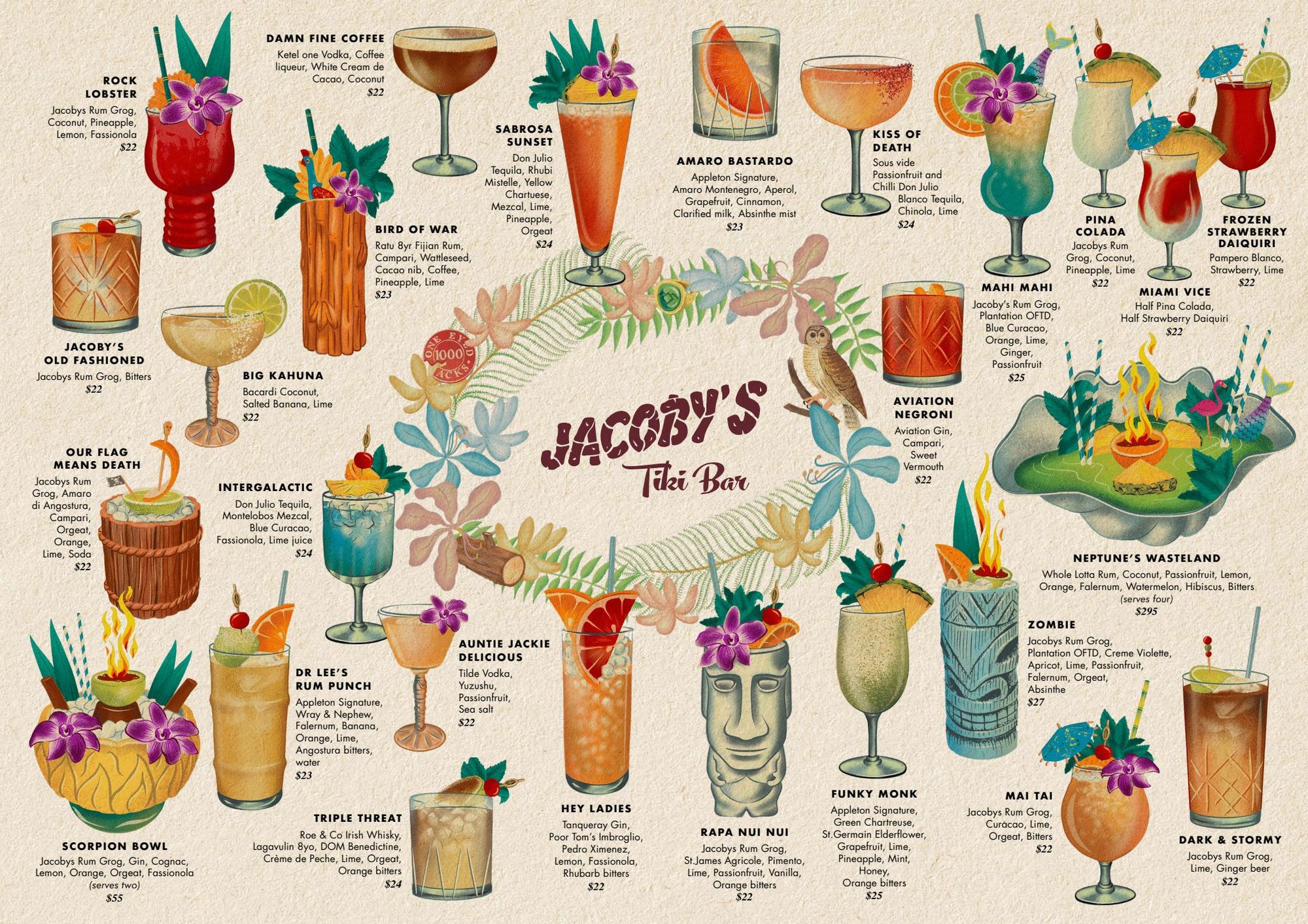This photograph showcases a rectangular, landscape-oriented menu for Jacoby's Tiki Bar, centered with the establishment's name in a prominent burgundy font. The off-white background provides a clean, elegant canvas for the vibrant drink illustrations that adorn the edges of the menu. Each tropical drink is meticulously detailed with its name and a list of ingredients beneath. These colorful concoctions are depicted in a variety of shades, including red, orange, purple, blue, yellow, teal, and green. Some drinks feature whimsical straws, while others are adorned with decorative flowers, embodying the festive and exotic essence of a tiki bar ambiance.